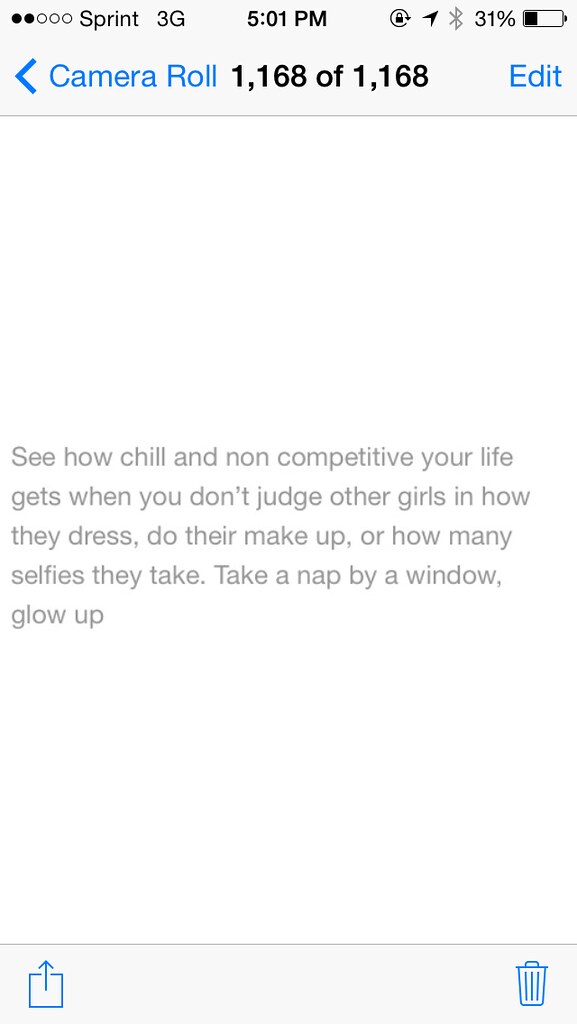The image is a detailed screenshot of an iPhone's camera roll interface. It showcases the screen at 5:01 PM with the Sprint 3G network and two out of five signal bars displayed, alongside icons for Bluetooth and location services, both of which appear grayed out. The battery life is at 31%. 

At the top left, it indicates that this view is within the Camera Roll, specifically showing item 1168 of 1168. A blue "Edit" button is positioned at the top-right corner. Centrally displayed on the screen is a motivational message in a light gray hue that reads: "See how chill and non-competitive your life gets when you don't judge other girls in how they dress, do their makeup, or how many selfies they take. Take a nap by a window, glow up."

Towards the bottom of the screen, there are two prominent icons: a square with an upward-pointing arrow symbolizing an upload or share function on the left, and a trash can icon for deletion on the right.